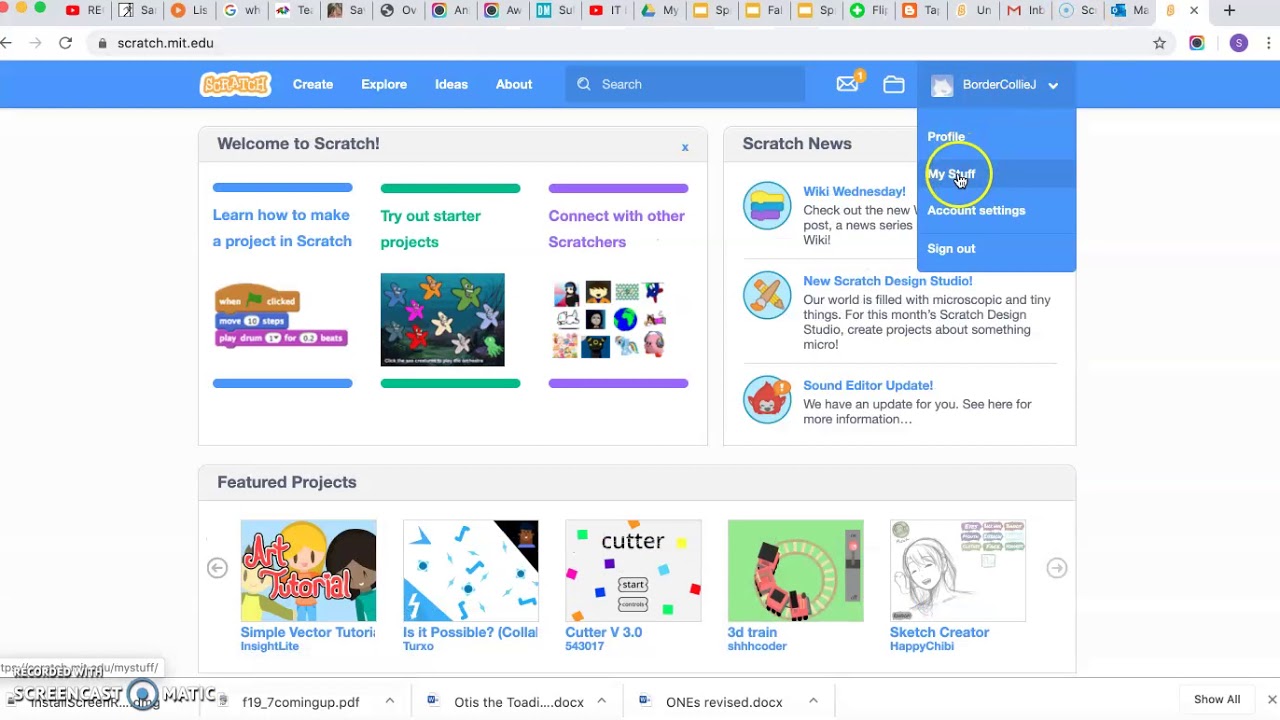This is a screenshot of a desktop displaying a web browser with over 20 tabs open. The active tab is navigated to [Scratch](https://scratch.mit.edu), as indicated by the URL in the address bar. Below the URL bar, a blue navigation bar spans the width of the page. On the left side of this bar, "Scratch" is prominently displayed in yellow text. The top menu features four white links: "Create," "Explore," "Ideas," and "About." Adjacent to these links on the right is a blue search bar.

Further to the right, there are icons for an envelope and a folder, followed by a user dropdown menu bearing the username "BorderCollieJ." The dropdown menu lists four options: "Profile," "My Stuff," "Account Settings," and "Sign Out." Notably, the "My Stuff" option is circled in yellow, drawing attention to it.